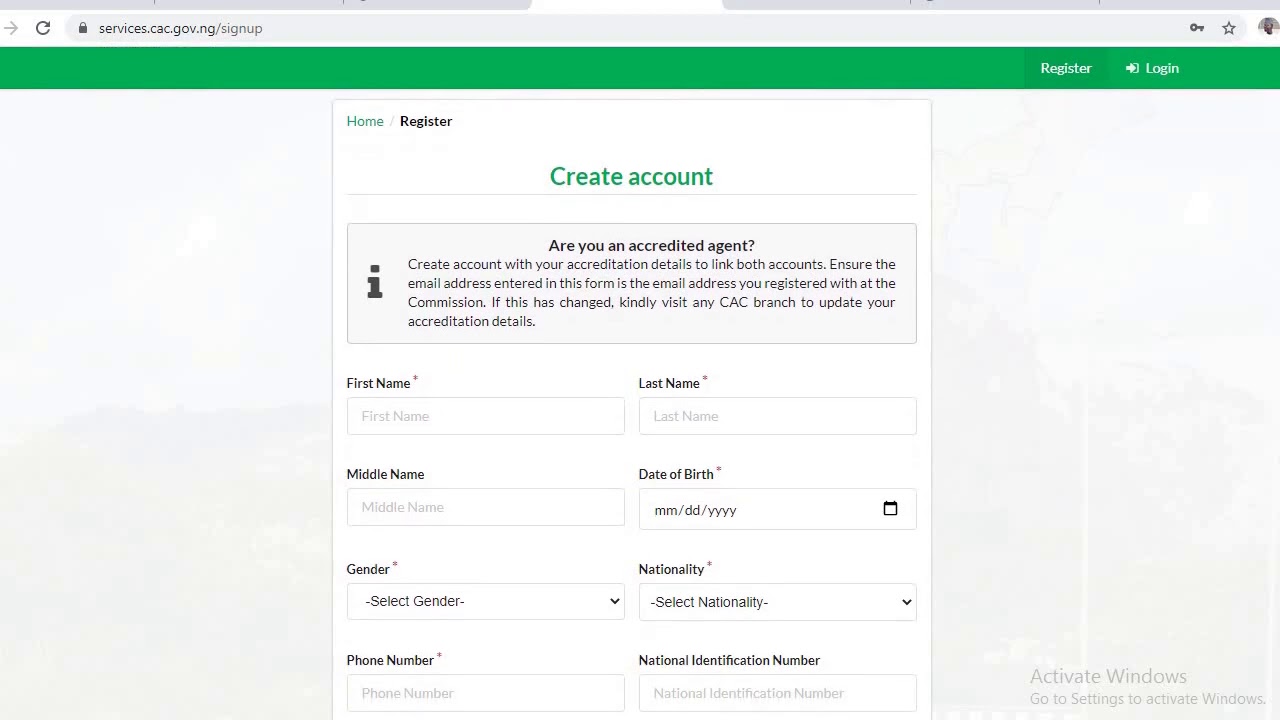This image is a screenshot from the website services.cac.gov.ng/sign-up. At the top of the webpage, there is a prominent green bar that spans its entire width, providing a visually appealing and consistent header. Located within this header are two essential buttons: "Register" and "Login," easily accessible for users.

Dominating the central portion of the webpage is a section dedicated to account creation. Here, users are prompted with a message: "Are you an accredited agent? Create an account with your accreditation details to link both accounts. Ensure the email address entered in this form is the email address you registered with at the commission. If this has changed, kindly visit any CAC branch to update your accreditation details."

Below this informative message, the form fields required for account creation are displayed. These fields include input boxes for first name, last name, middle name, date of birth, gender, nationality, phone number, and national identification number, catering to a comprehensive identity verification process.